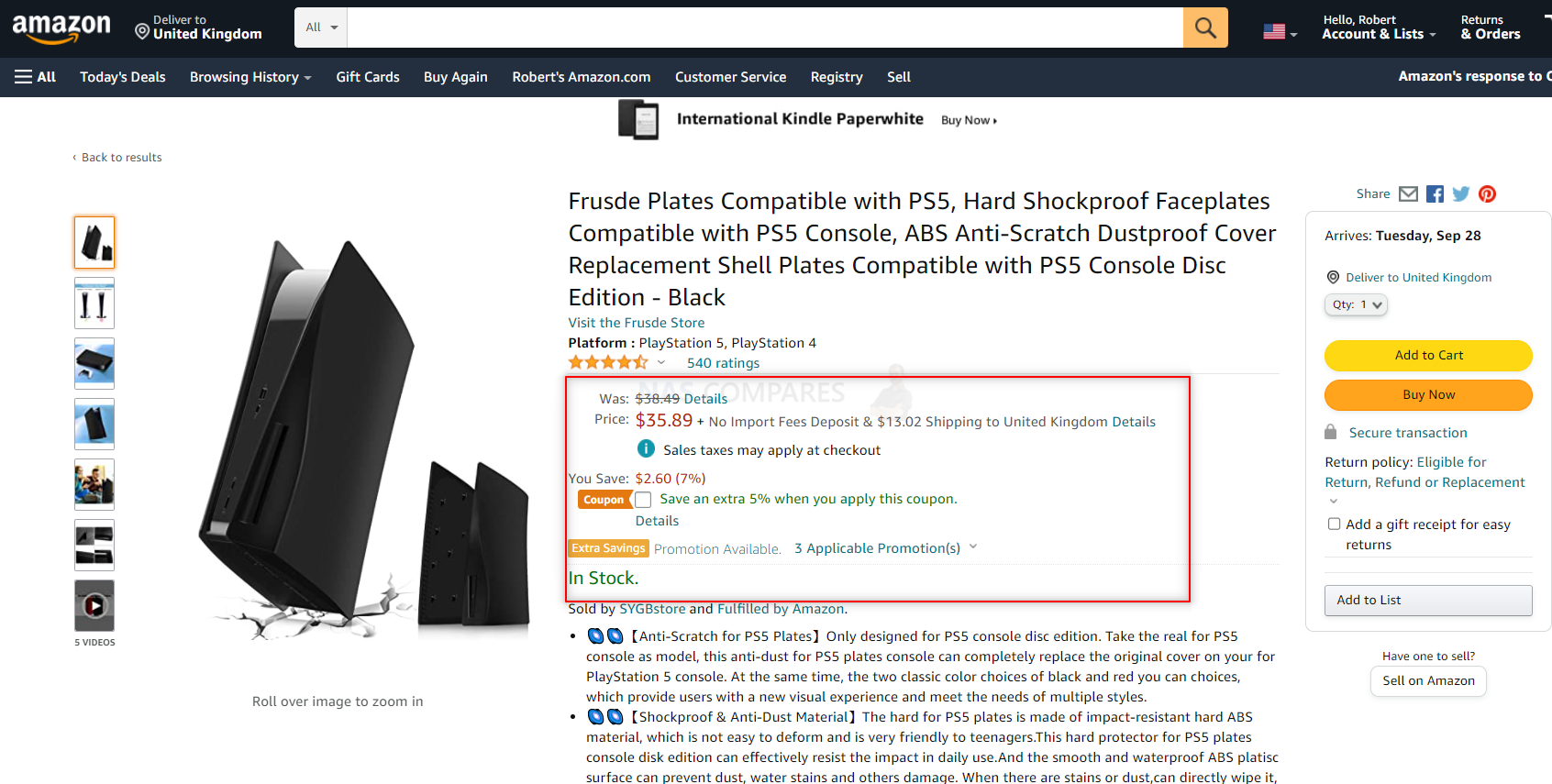### Detailed Caption of Amazon Product Page for PS5 Plates

This image displays a detailed view of an Amazon product listing page. At the very top, the page reads "Amazon" with the Amazon logo prominently positioned on the top left. To the right of the logo, there's a message that reads "Delivered to United Kingdom."

Below the header, there's an empty search bar with a magnifying glass icon indicating a search function. Adjacent to the search bar, there is a small icon of the USA flag and text indicating "Hello Robert," followed by account options such as "Account & Lists," "Returns & Orders." 

Further down, a navigation bar presents various categories including "Today's Deals," "Browsing History," "Gift Cards," "Buy Again," "Robert's Amazon.com," "Customer Service," "Registry," and "Sell."

The main content of the page features an image of a black PS5 with black faceplates. To the left of this main image are several smaller images showing different angles and aspects of the product. 

To the right of the main image, the product is described as "Frusty Plates Compatible with PS5 Hard Shockproof Faceplates Compatible with PS5 Console ABS Anti-Scratch Dust Proof Cover Replacement Shell Plates Compatible with PS5 Console Disc Edition - Black." The product is sold by "Frusty Store" and it is compatible with both PlayStation 5 and PlayStation 4 platforms. The product has a rating of four stars out of five from 540 ratings.

Listed beneath the title, the price marked in red reveals a discount: it was £38.49, now £35.89. There's no import fees deposit, and shipping to the United Kingdom is £13.02. Retail taxes may apply at checkout. A note indicates that you save 2.67%, and there's an option to save an additional 5% by applying a coupon, highlighted in blue.

The product is shown as in stock with a red square indicating availability. It is "Sold by SYGB Store and fulfilled by Amazon." The description adds details about the product: it's anti-scratch and designed specifically for the PS5 console disc edition. Made of impact-resistant hard ABS material, it is also shockproof, anti-dust, and designed to withstand daily use. The hard ABS plastic surface is smooth and waterproof, protecting against dust, water stains, and other damage.

Above the product details, social sharing buttons are available for email, Facebook, Twitter, LinkedIn, and Pinterest. 

To the right, there is a section for ordering information stating that the product arrives by Tuesday, September 28. Quantity can be adjusted via a drop-down menu. There are two buttons: a yellow "Add to Cart" button and an orange "Buy Now" button, indicating secure transactions. Additional options include a checkbox for adding a gift receipt for easy returns and an "Add to List" button.

At the bottom of the product options, it reads "Have one to sell? Sell on Amazon," inviting potential sellers to list their items.